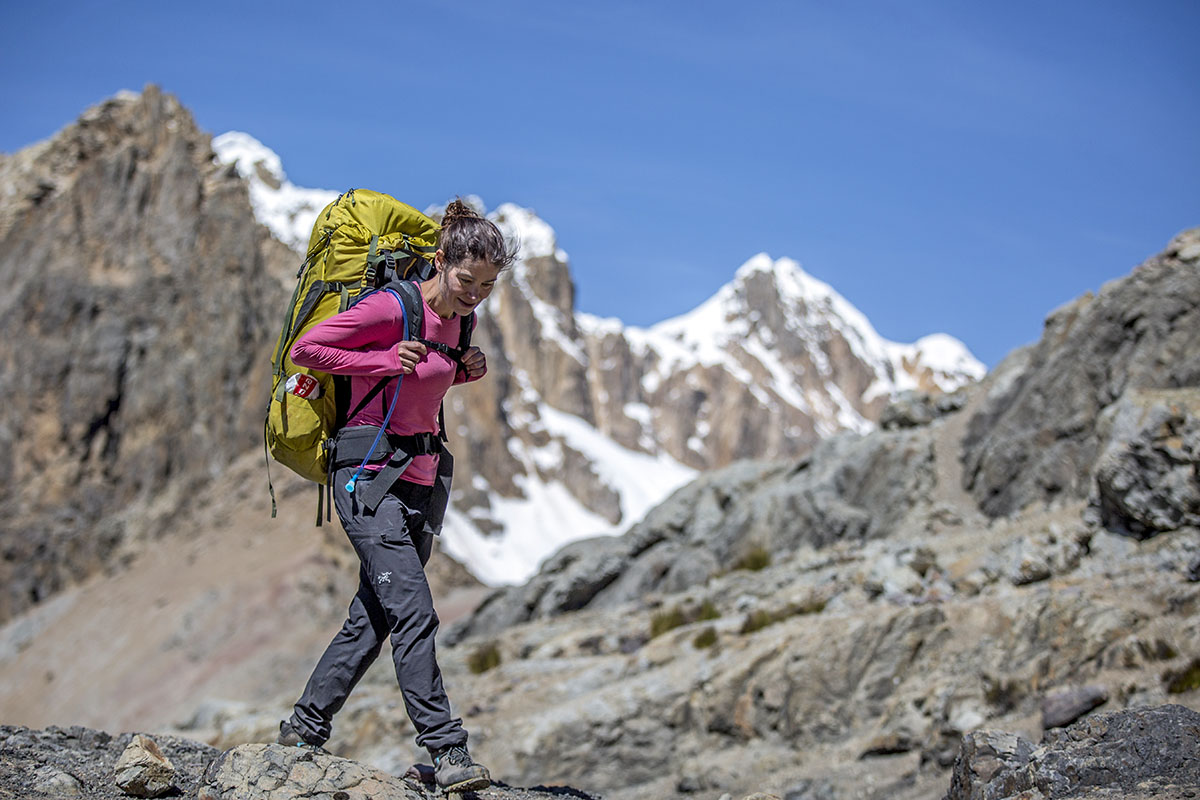In this photograph, a female hiker is captured navigating a mountainous terrain with the sun shining brightly above. She wears a long-sleeve pink shirt and dark gray cargo pants, with light brown hiking boots equipped for rugged paths. Her dark brown hair, tied up in a ponytail, stays out of her face as she looks downward, paying close attention to her steps. She carries a large, heavy-duty yellow backpack strapped securely around her waist and chest, with what appears to be a bag of chips sticking out. An additional strap, resembling a lanyard, is looped around her arm, possibly holding a compass. The background showcases a stunning, dual-layered mountainous landscape with one slope descending to the left and a more distant peak capped with snow against a clear blue sky, sloping in the opposite direction.